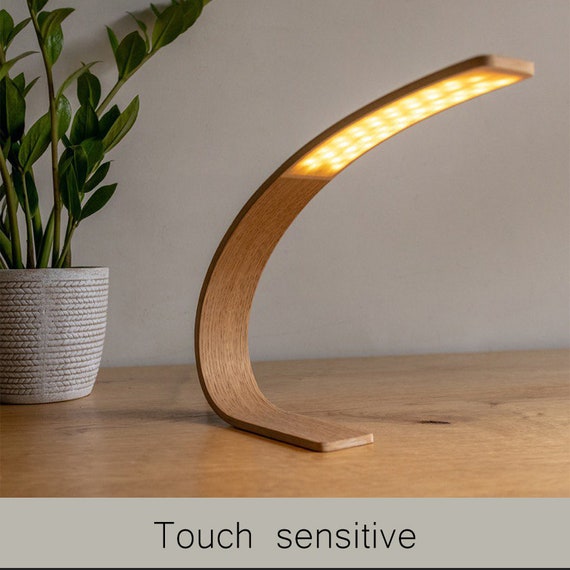The photograph features a modern, uniquely designed desk light, with a sleek, curved wooden structure resembling a C-shape or an arch, situated on a wooden table. The curved wooden plank has an upward curve to the right, with a series of golden LED lights embedded along the upper 30-40% of its inner curve. This touch-sensitive light, which likely operates with a concealed battery due to the lack of visible cords, is placed on a wooden countertop that harmonizes with the light's material. To the left of the light is a white ceramic flower pot with horizontal braid-like etchings, housing a fresh, green plant with leaves extending upwards. The setting is backed by a light gray wall, and a gray banner at the bottom of the image contains the black text "touch sensitive," highlighting the feature of the lamp. The overall style of the image is photorealistic.